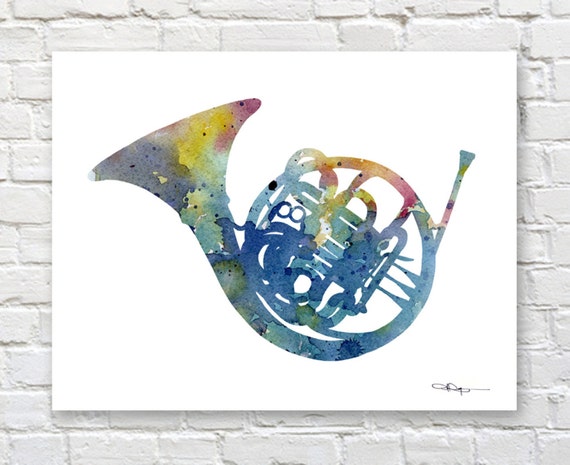The image depicts a vibrant watercolor painting of a French horn set against a white, brick-patterned wall. The painting, set on a white field nearly filling the frame, showcases the instrument lying on its back, with the bell extending towards the upper left and the mouthpiece reaching to the upper right. The intricate tubing and valves are centrally positioned. The French horn is adorned with a whimsical array of colors, including reds, yellows, blues, purples, greens, and oranges, creating an abstract and dynamic visual. The painting is signed in the bottom right corner.